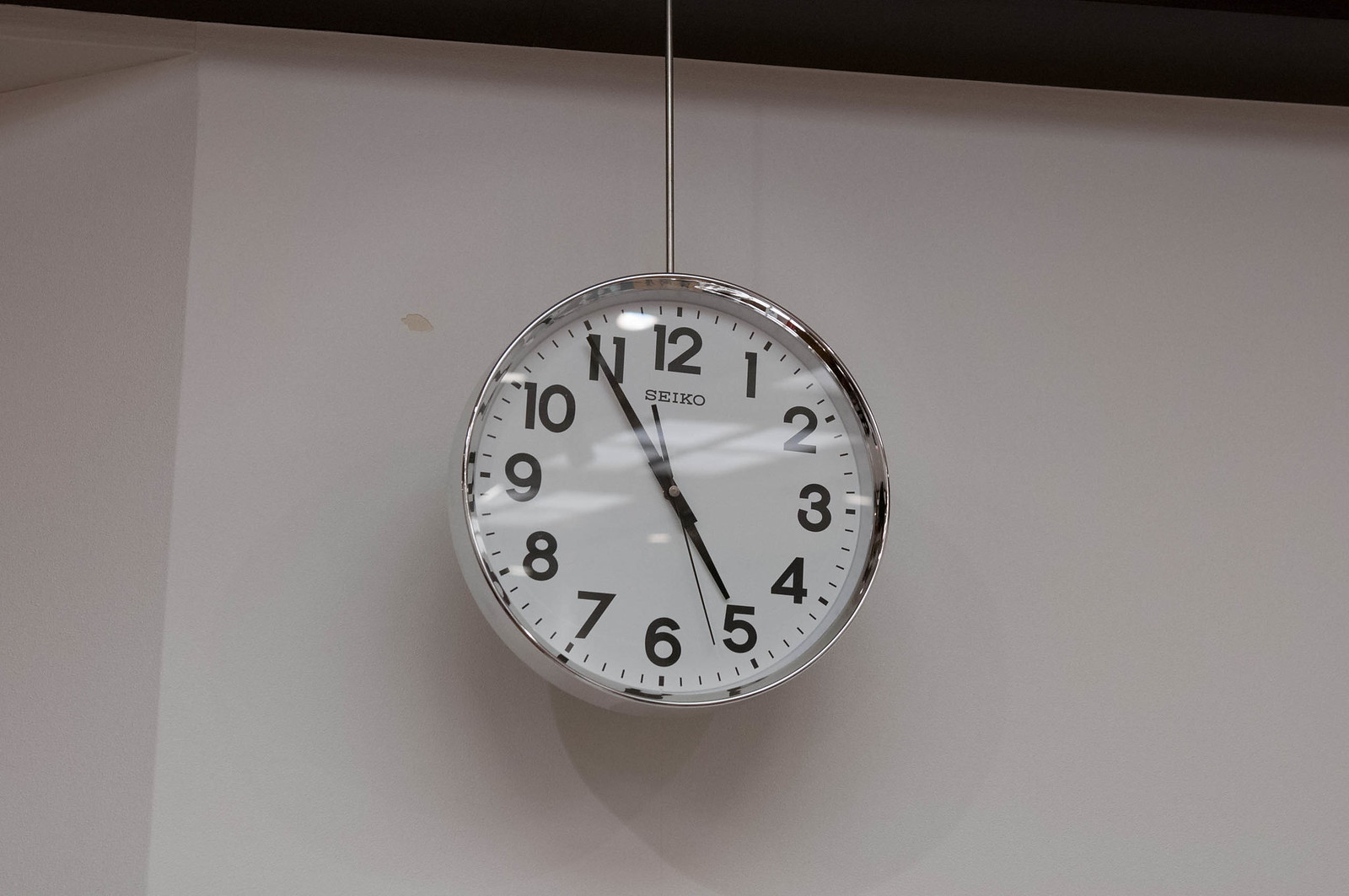In this black-and-white photographic image, a classic, simple wall clock is prominently displayed against a white wall with a corner to the left. The clock, which appears to be hanging from the ceiling by a rigid metal rod, is adorned with a reflective silvery metal housing. The clock face is white, featuring black Arabic numerals and black minute, hour, and second hands, all anchored at the center by a small gold piece. The brand name "Seiko," spelled S-E-I-K-O, is clearly visible on the face of the clock. The time shown is approximately 4:54, with the second hand precisely at 27 seconds. Above, the ceiling is dark, contrasting with the white wall. Noteworthy details include a faint red smudge just to the left of the clock, adding a subtle touch of color to the otherwise monochromatic setting. The clock exudes a timeless, functional design, seamlessly integrating into its minimalist surroundings.